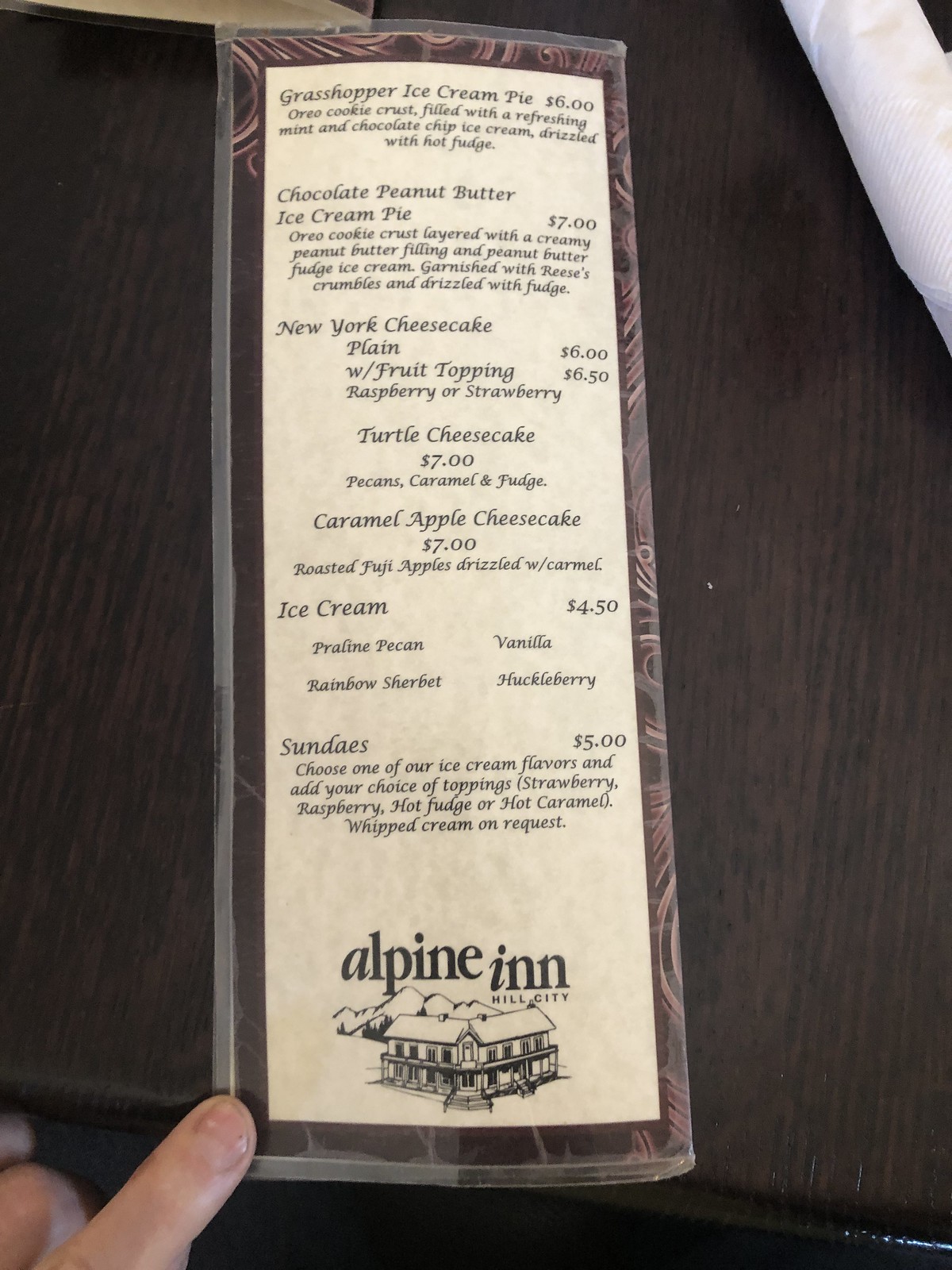This is a photo displaying a compact, rectangular dessert menu from Alpine Inn, Hill City. The menu begins with a feature item, the Grasshopper Ice Cream Pie, priced at $6, which includes an Oreo cookie crust filled with refreshing mint and chocolate chip ice cream, all drizzled with hot fudge. 

Next, the Chocolate Peanut Butter Ice Cream Pie is listed at $7. It boasts an Oreo cookie crust, layered with creamy peanut butter filling and peanut butter fudge ice cream, garnished with Reese's crumbles and drizzled with fudge.

The menu continues with a New York Cheesecake, offered plain for $6, or with a fruity topping (raspberry or strawberry) for $6.50. Following that is the Turtle Cheesecake, priced at $7, featuring a combination of pecans, caramel, and fudge.

Another option is the Caramel Apple Cheesecake for $7, which includes roasted Fuji apples drizzled with caramel. The menu also lists various ice creams at $4.50, including praline pecan, rainbow sherbet, vanilla, and huckleberry.

Additionally, sundaes are available, where you can choose one of the ice cream flavors and add toppings such as strawberries, raspberry, hot fudge, or hot caramel. Whipped cream is available upon request.

At the bottom of the menu, there is a small sketch of a building, along with the name "Alpine Inn Hill City."